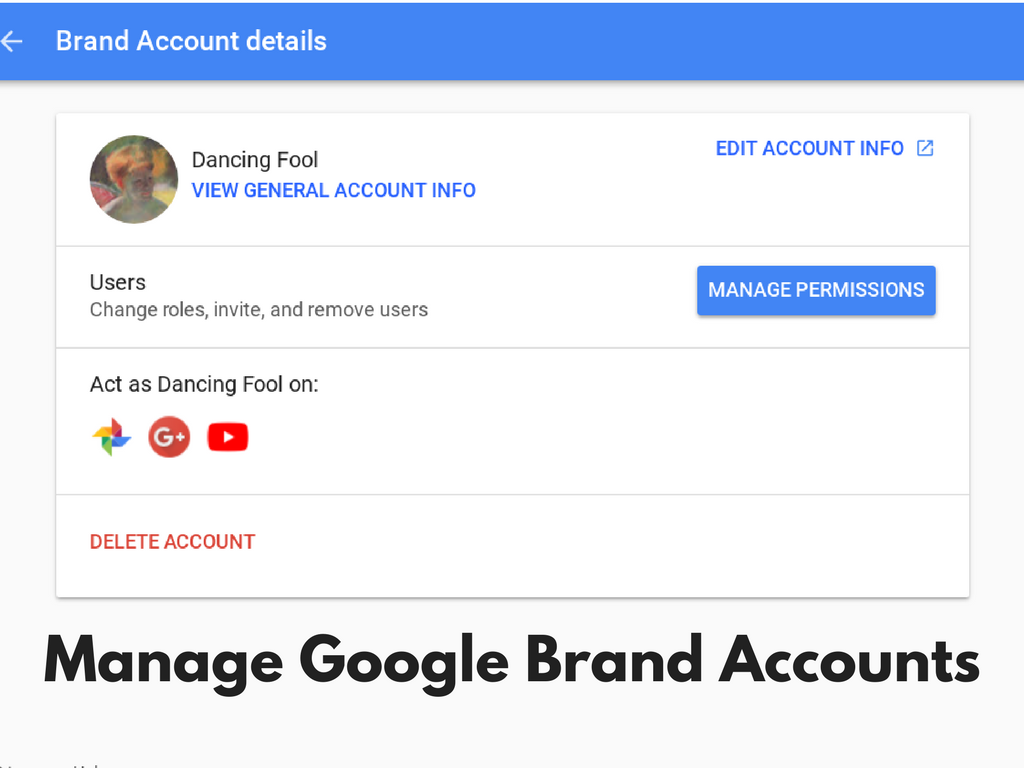The image displays a web interface for managing a Google brand account. At the top, there's a blue banner with shadowed edges. The top-left corner of this banner includes the label "Dancing Fool" and offers options to view general account info, while the top-right corner provides a link to edit account info. Below this banner, there are several options listed: "Users," "Change Roles," "Invite and Remove Users," and "Manage Permissions."

A prominent blue rectangle in the main interface area reads "Manage Permissions" and allows users to act as the brand "Dancing Fool." Below this, a red circle encloses the Google+ logo, with YouTube icons adjacent to it and an option to delete the account. There is also a section to manage Google brand accounts. The overall background is white, and the interface includes shadowed lines and divisions for clear segmentation.